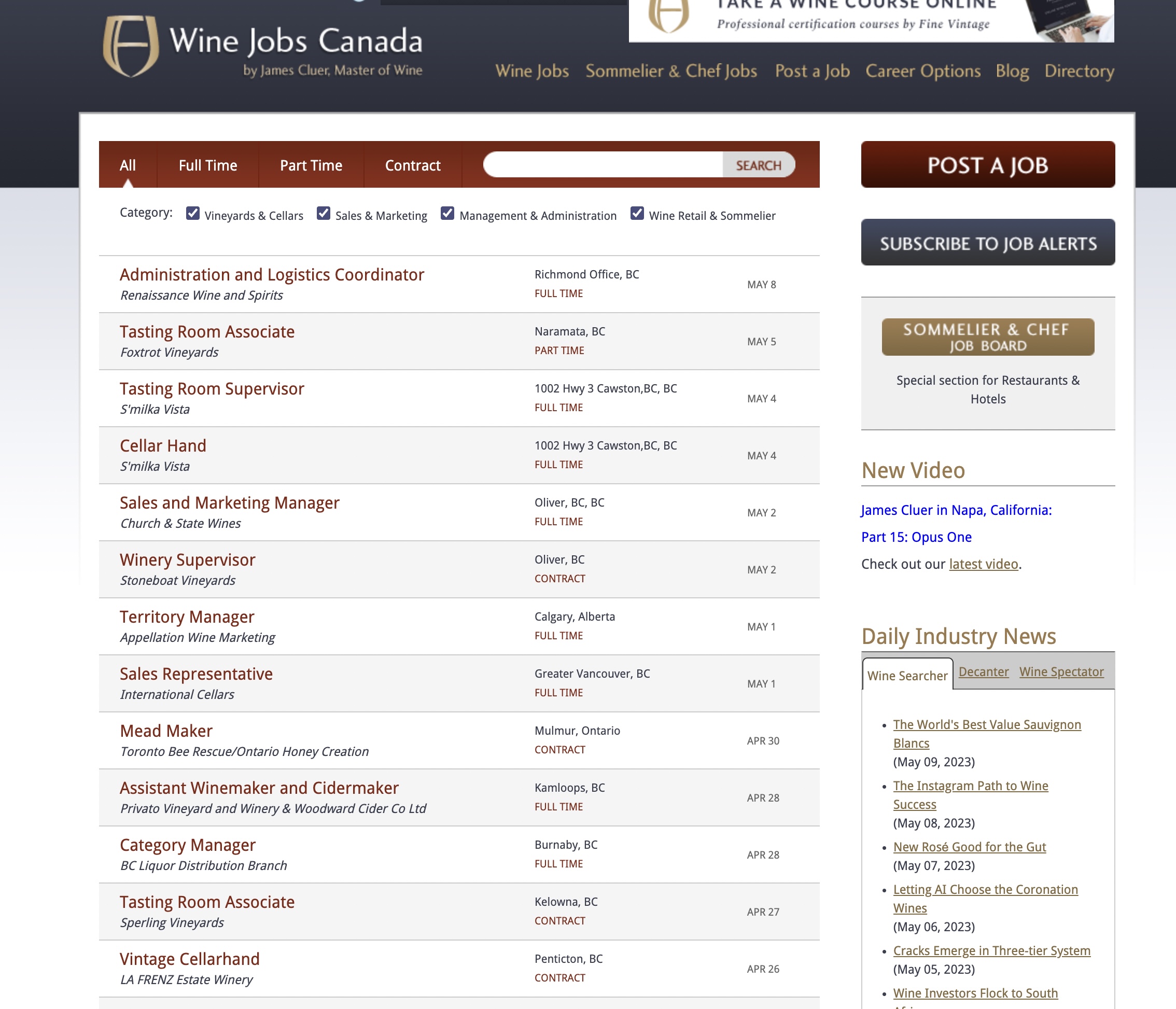This image features a sleek, professional design with a dominant black background, accentuated by a gold wine glass icon and elegant gold lettering. At the top, it reads "Wine Jobs Canada" by James Kluwer, Master of Wine, establishing both credibility and focus. The gold text further elaborates on navigation options: "Wine Jobs," "Sommelier and Chef Jobs," "Post-A-Job," "Career Options," "Blog," and "Directory."

Beneath this, the image transitions to a white background highlighted with a rich maroon accent. The top section includes a maroon arrow pointing upwards towards the word "All" in white lettering, followed by options "Full-Time," "Part-Time," and "Contract." Below these options, a search engine bar is prominently featured, with the word "Search" in maroon text.

Continuing downward, the image displays various job categories in blue boxes with white check marks, including: "Vineyards and Cellars," "Sales and Marketing," "Management and Admission," and "Wine and Retail Sommelier." 

In a structured, list-like format, additional job titles are displayed in maroon text: "Administration and Logistics Coordinator," "Tasting Room Assistant," "Tasting Room Supervisor," "Cellar Hand," "Sales and Marketing Manager," "Winery Supervisor," "Territory Manager," "Sales Representative," "Mead Maker," "Assistant Wine Maker and Cider Maker," "Category Manager," "Tasting Room Associate," and "Vintage Cellar Hand."

The right column provides location details and employment types in practical information like "Richmond, BC, Full-Time," "Near Rana, BC, Part-Time," and addresses such as "102 Highway 3 Crossing," complete with owner names and relevant dates. This comprehensive layout effectively caters to individuals seeking detailed information on wine-related employment opportunities in Canada.